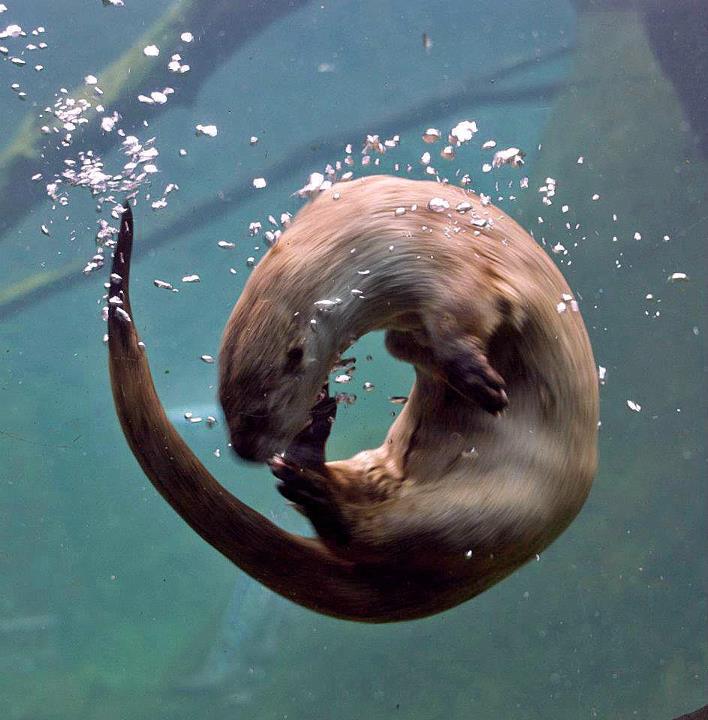This drawing or painting depicts an adorable sea otter, gracefully curled into a ball as it swims underwater. The otter, with its brown-gray fur, is positioned in a circular motion, with its head nestled close to its back feet and its long tail arching over its head, almost resembling a yin and yang symbol. Its eyes are peacefully closed, giving the impression that it might be sleeping or comforting itself. The creature's two front paws are extended outward on either side of its body, adding to the fluidity of its pose. Surrounding the otter are bubbles, indicating its underwater environment, possibly from its breathing. The blurred background, painted in shades of blue, teal, and green, is filled with indistinct tree branches, suggesting a natural underwater habitat. The overall scene illustrates the otter's playful nature and its comfort in the aquatic surroundings.